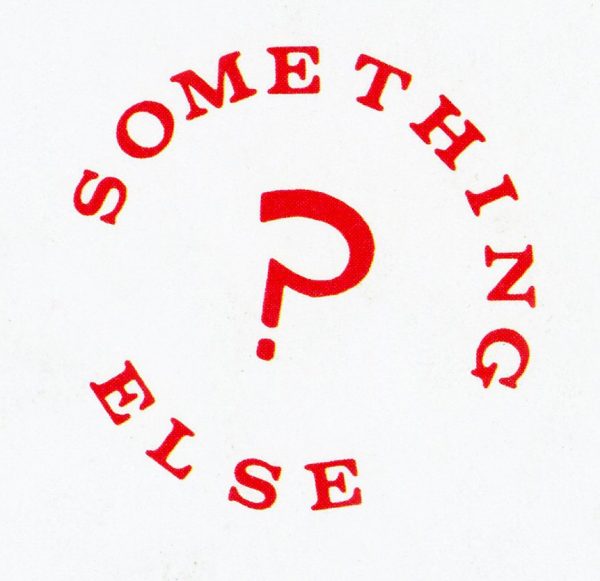Centered on a plain white background, the image features a bold, circular logo with the text "SOMETHING ELSE" surrounding a large, cartoony question mark. The text, written in a formal serif font, is in all capital letters and a bright orangey-red color. "SOMETHING" arches around the top right side of the question mark, while "ELSE" curves around the bottom left, together creating a ring-like formation. The question mark itself, in the same red hue, is prominently placed in the center, giving the appearance of a cohesive sticker or decal design that stands out against the stark white background. The arrangement is slightly off-center, with "SOMETHING" aligning more with the top right and "ELSE" with the bottom left.